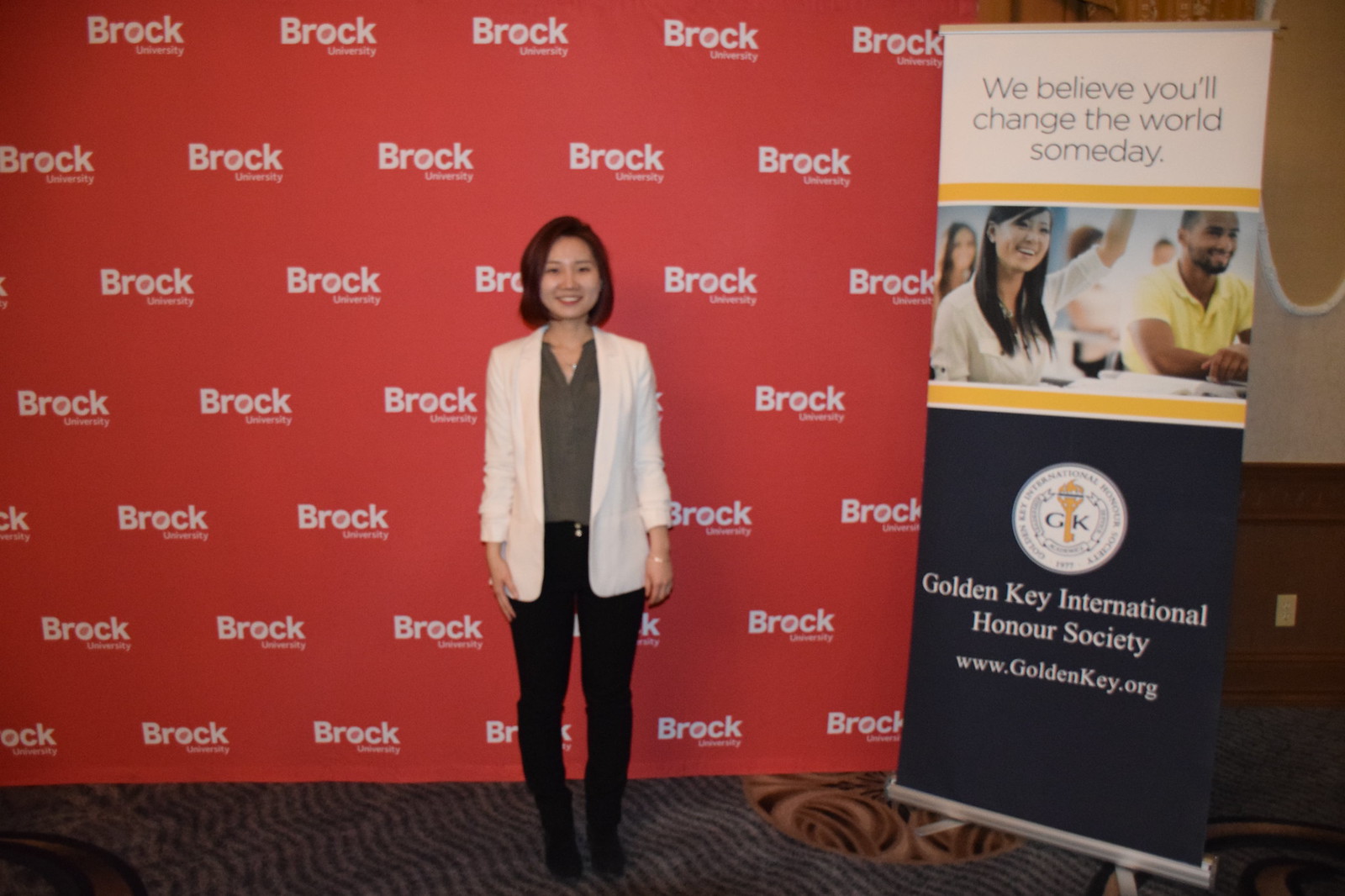The image depicts an Asian woman with long brown hair, standing straight and smiling at the camera with her arms at her sides. She is dressed in a white jacket, gray shirt, and black pants. The backdrop is a red wall repeatedly featuring the name "Brock" in varying sizes, indicative of Brock University. To her right stands a tall banner with the message, "We believe you'll change the world someday," at the top against a white background, followed by a horizontal gold stripe beneath which there is an image of university-aged students. Below this, on a black background, the banner displays the emblem of the Golden Key International Honor Society, described as the letters "GK" with a golden key symbol surrounded by laurel branches. The text "Golden Key International Honor Society" along with the website "www.GoldenKey.org" is clearly visible in white lettering. The woman stands on a gray, wavy-patterned rug, completing the well-composed and professional scene designed for photo opportunities at the event.